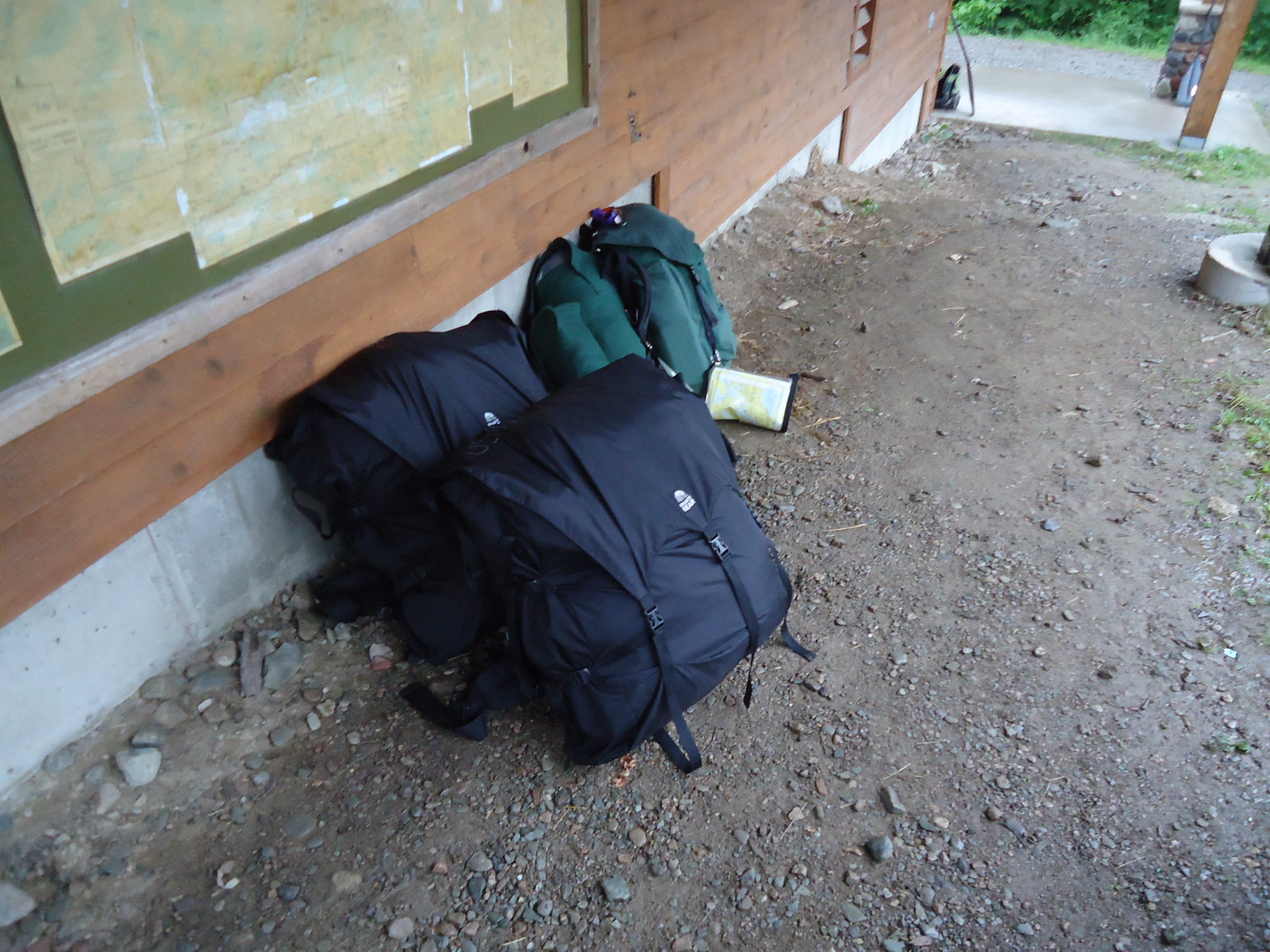In this outdoor color photograph taken during the daytime, three backpacks are seen leaning against the side of a partially finished building. The ground in front of the building is rocky dirt, with some cement visible in the background, possibly part of a sidewalk. The building has a concrete base with brown horizontal wood paneling above it. An old wooden frame, containing a map on a green background, is attached to the wall, suggesting this could be a hiking area.

The backpacks include two dark blue ones, one of which leans directly against the building while the other leans against the first blue backpack. Next to them, a dark green backpack also leans against the building. The scene suggests a resting spot for hikers, given the rugged appearance of both the ground and the building. On the right side of the frame, there is a glimpse of grass growing, indicating an area transitioning from the rocky dirt surface.